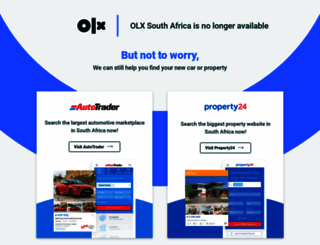The image features a split background with light blue occupying the top and bottom sections and a large dark blue semi-circle dominating the center. At the top, the caption "OLX South Africa is no longer available" is displayed with a small blue line, followed by a message in blue print encouraging users not to worry and offering alternatives to find cars or properties.

On the left side, there's a white and blue box featuring the AutoTrader logo, with "Auto" in red and "Trader" in black. A red and blue line accentuates the logo. This section invites users to "Search the largest automotive marketplace in South Africa now" and includes a 'Search' button. Below it, there is an image of a red car set against a blue background, which provides additional information in a white box underneath.

On the right side, another white and blue box features the Property24 logo, with "Property" in blue and "24" in red. It encourages users to "Search the biggest property website in South Africa now," accompanied by a 'View Properties' button. Adjacent to this, there's an inset containing an image of a house with orange and blue elements on top and white on the bottom. Additionally, there's a blue box featuring a white box inside it and a red button at the bottom.